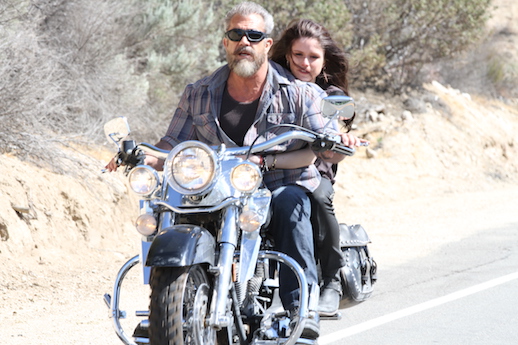The photo captures an older man and a younger woman riding a motorcycle on what appears to be a highway in an arid, desert-like environment with sparse shrubbery and rocks in the background. The man, who is driving, has white hair, a white beard, and is dressed casually in a plaid jacket over a black t-shirt, jeans, and sunglasses. The woman sitting behind him, with her arms around his waist, has long brown shoulder-length hair, black jeans, and cowboy boots. The motorcycle, which is primarily silver with a black fender and black tires, has its headlights on, possibly for safety, and is seen coming directly toward the viewer. The bright glare of sunlight adds to the overall impression of an outdoor, desert setting.